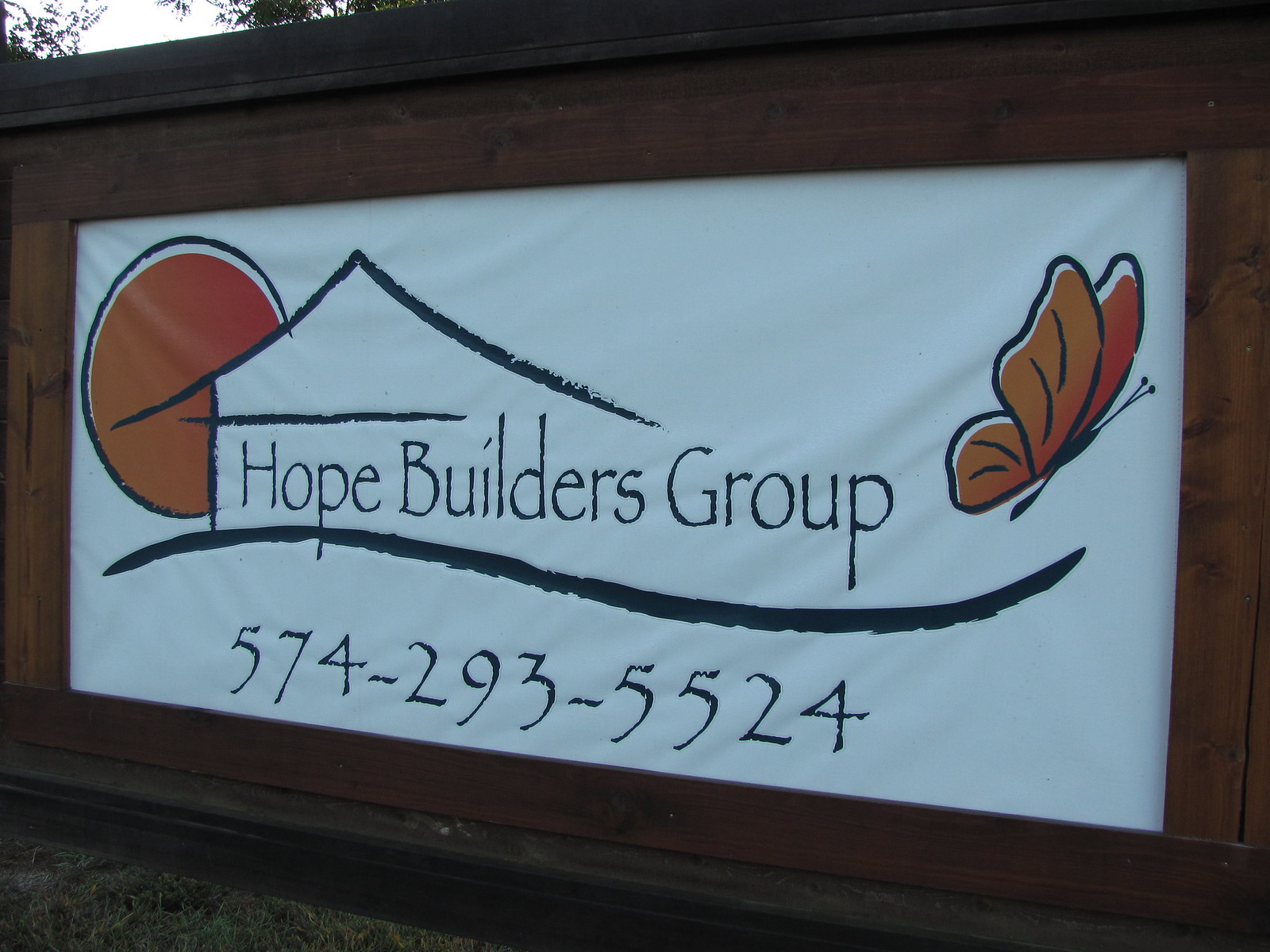A close-up image showcases an advertisement banner mounted within a wooden frame, part of a larger wooden structure. In the background, the top left corner reveals the bright sky and green leaves from nearby trees, while the bottom left corner shows a patch of grass. The banner itself is composed of fabric and features a detailed design: an outlined picture of a house with an orange sun rising behind it, an orange butterfly, and a small hill. Inside the house's outline, in black text, the company name "Hope Builders Group" is prominently displayed. Below the company name and bisected by a curved horizon line, the phone number "574-293-5524" is also printed. The banner's plain white background highlights the vibrant and structured elements of the advertisement.